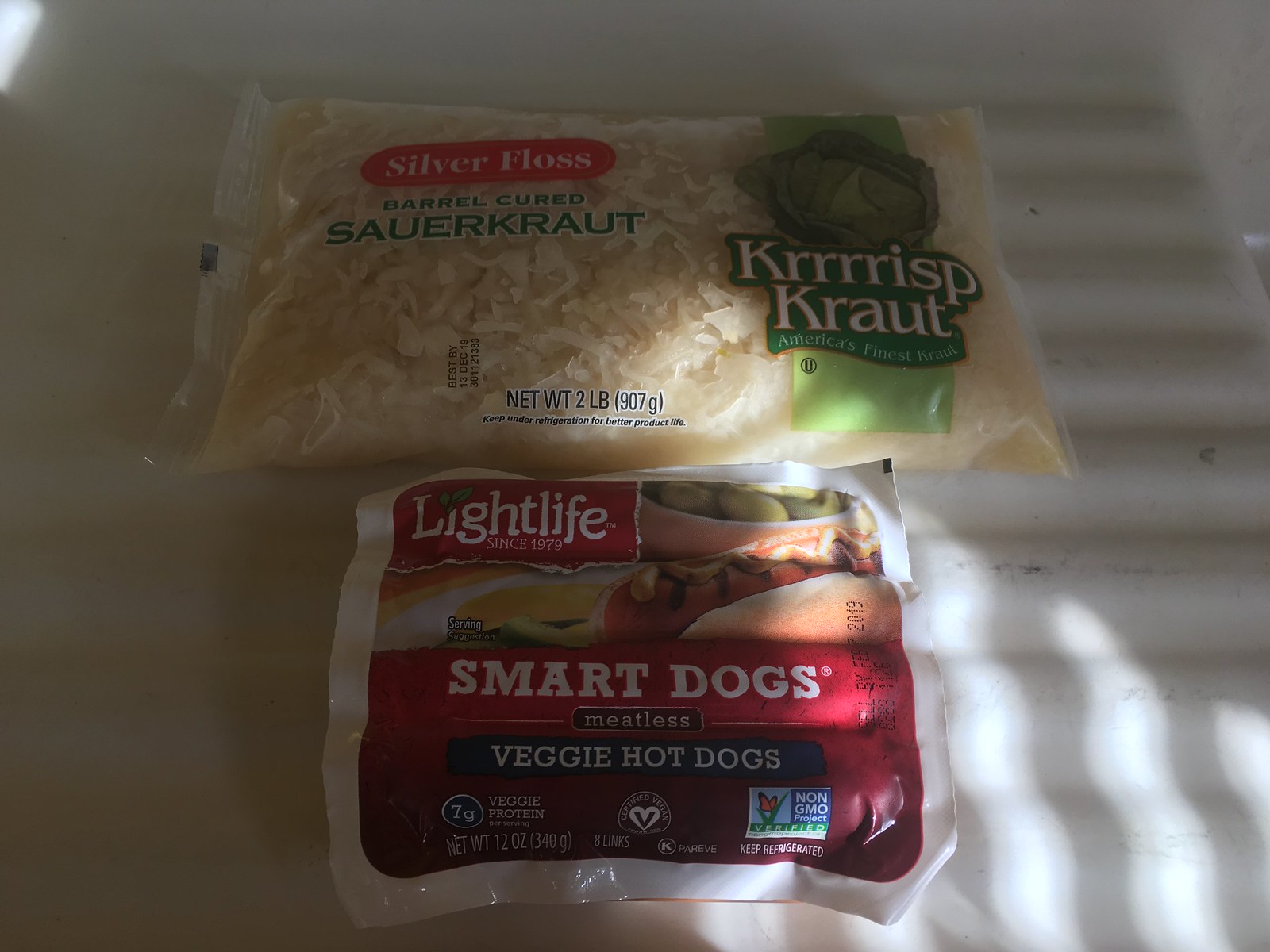The image depicts two food packages resting on a white, wavy-contoured surface, which appears to be either a refrigerator shelf or a tabletop. On the right side of the surface, there are black marks, possibly from wear or staining. The first package, positioned on the left, is a rectangular clear bag containing tan-colored sauerkraut. The bag is labeled "Silver Floss Barrel Cured Sauerkraut" in green text, with additional phrases like "Crisp Kraut" and "America's Finest Kraut." There is also an image of a plant on the packaging. The second package, located on the right, is red and white and contains "Smart Dogs Meatless Veggie Hot Dogs." This packaging includes the brand name "Lightlife" with the founding year "Since 1979," and highlights that each serving contains "7 grams of veggie protein."